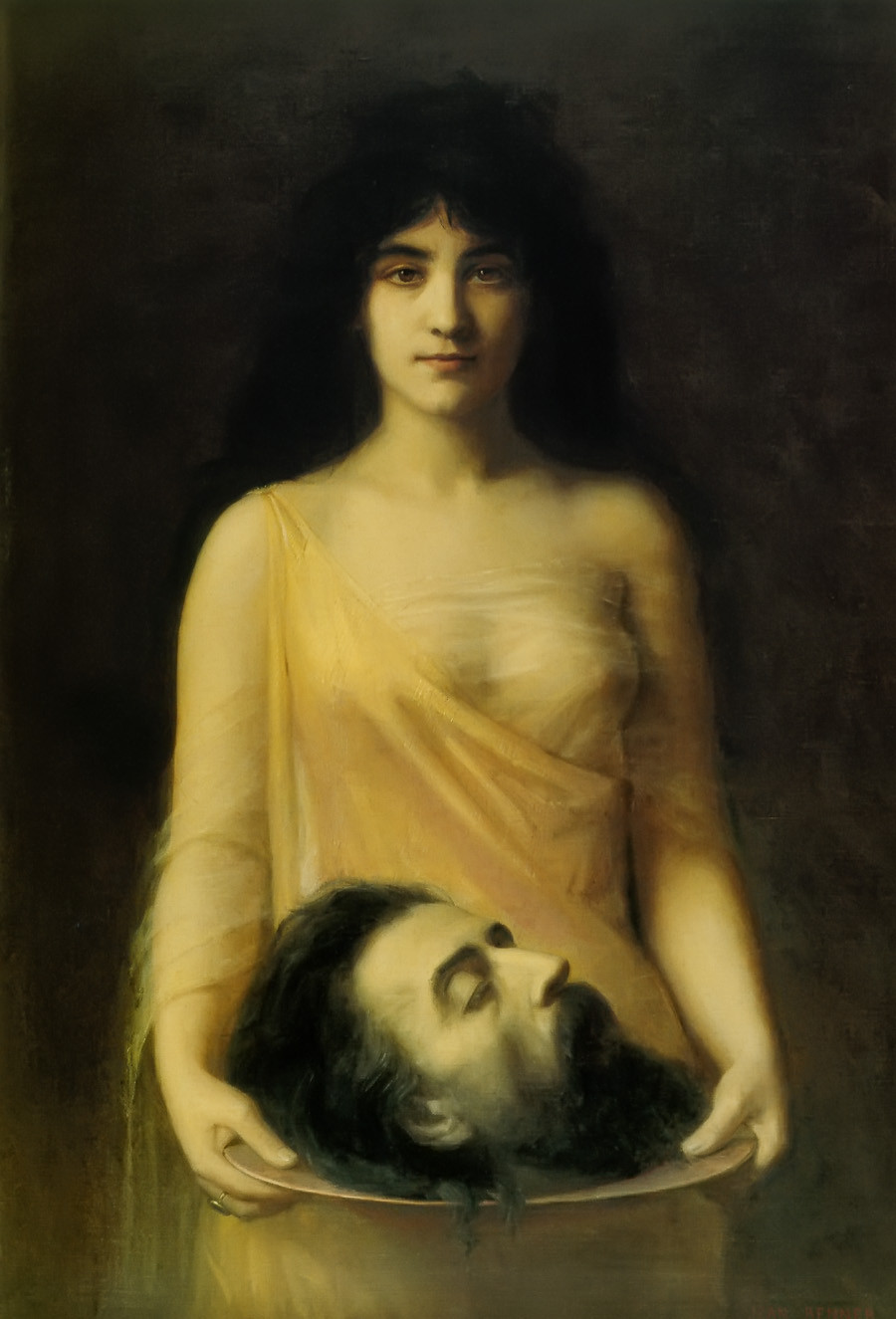The image depicts a woman, evocative of classic representations of Salome with John the Baptist's head. She stands holding a round platter firmly in both hands, displaying a man's severed head, with dark hair and a beard, his eyes closed. The woman is dressed in a loose-fitting, light yellow dress that drapes gently around her, partially covering her. Her facial expression is notably plain—neither sad nor joyous, but neutral, as she gazes directly at the camera. Her dark hair frames her face, which appears partly shadowed, adding to the overall dramatic ambiance of the painting. The background is a deep, shadowy brown at the top, transitioning into blurry hues of brown and yellow towards the bottom, giving the entire scene a somber, almost ominous tone. The colors predominantly used in the image are yellows and browns. The woman is of average build, not overly thin nor heavy, with a presence that commands attention within the composition.